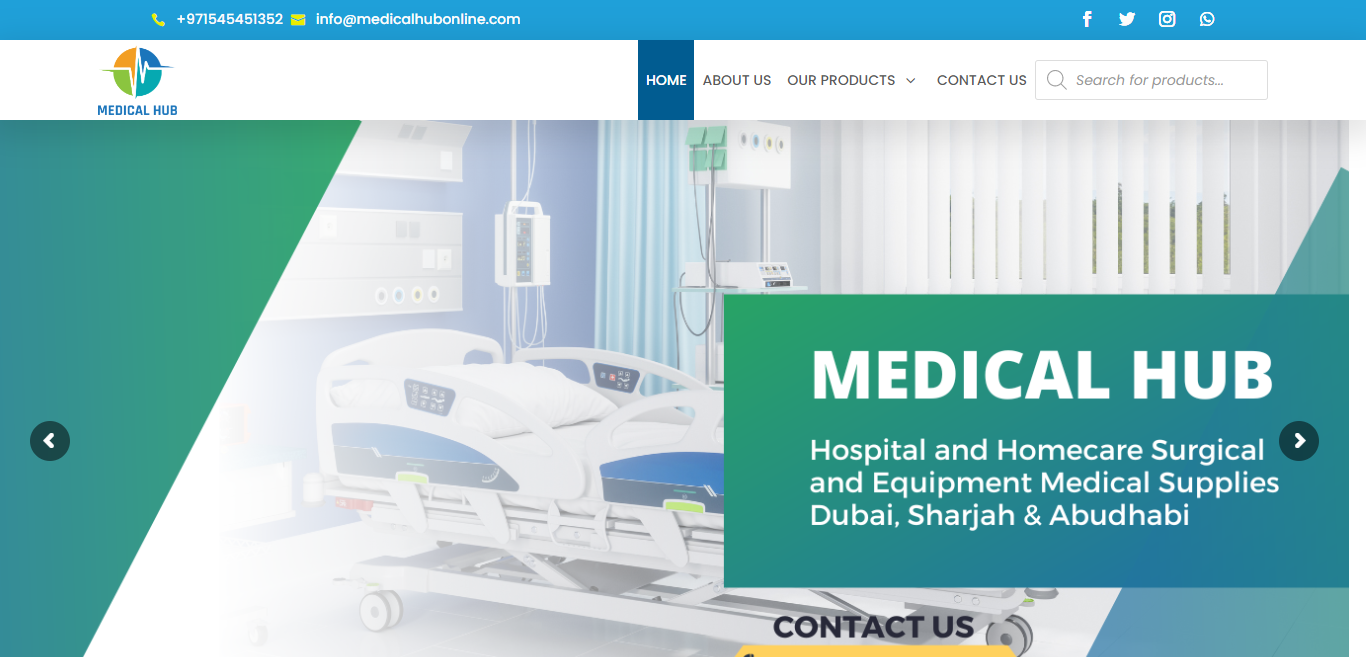Screenshot of the Medical Hub website featuring a central visual of an up-and-down heartbeat graphic over a multicolored circular background. The circle is divided into four segments: yellow at the top, dark blue on the right, light green on the bottom left, and aqua on the bottom right. Below the graphic, the text "Medical Hub" is displayed prominently.

The website header includes navigation options: "Home" highlighted with a blue background, indicating the current page, followed by "About Us," "Our Products" with a dropdown arrow, "Contact Us," and a search text box featuring a magnifying glass icon with the placeholder "Search for products."

Social media icons for Facebook, Twitter, Snapchat, and an unidentified platform are visible. The background image depicts a hospital room with a hospital bed, machinery, and blinds, emphasizing a modern and connected medical environment. Overlaying the image, white text on a green-aqua background reads "Medical Hub, hospital and home care, surgical and equipment, medical supplies, Dubai, Sharjah, and Abu Dhabi." Below the bed, in black letters, the text "Contact Us" is visible.